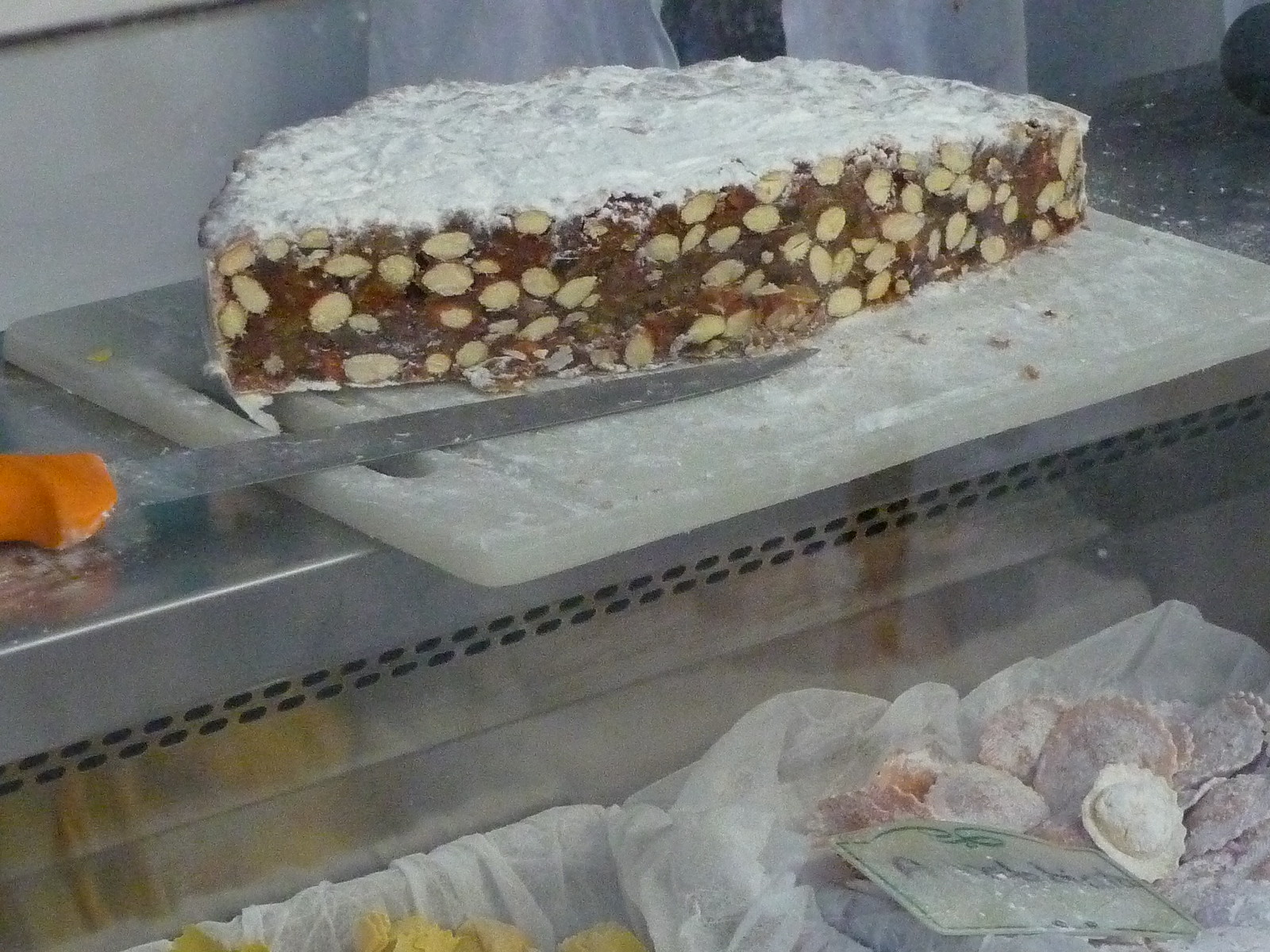The photo captures a detailed view through a display case, featuring an assortment of food items on a stainless steel shelf. On the top shelf, a large cutting board, dusted with powdered sugar, prominently displays a half-circle shaped cake or Italian dessert. This confection is coated in white sugar and its exposed cross-section reveals a brown interior studded with cream-colored nuts and possibly fruits, indicative of a rich, nutty filling. A long knife with an orange handle rests on the cutting board amidst a scattering of crumbs. Below, in cheesecloth-lined baskets, are an array of fresh pasta. The left basket contains typical yellow pasta, while the right basket showcases a colorful mix, likely ravioli, made with ingredients like spinach and carrots, evident from their orange and yellow hues. The reflection on the display glass adds a touch of realism to the scene, highlighting the vibrant and enticing food items within.